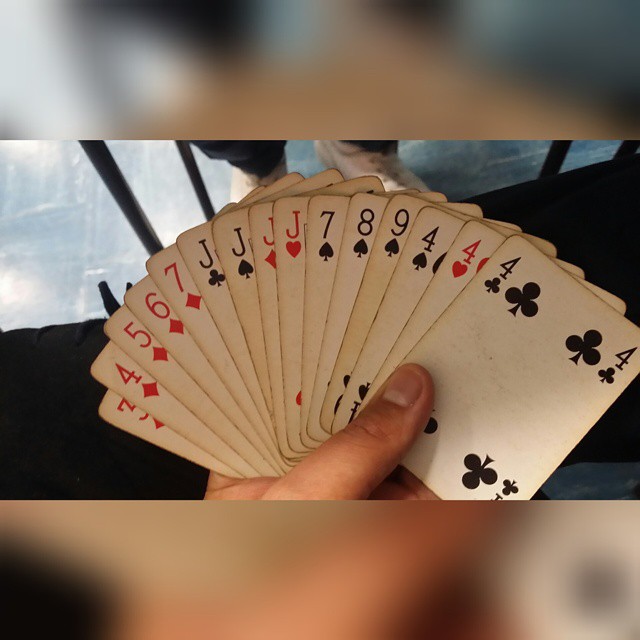A close-up image depicts a man holding a fanned-out hand of 15 playing cards. His thumb is positioned over the cards, with his fingers supporting them from behind. The cards are displayed in sequence from left to right: 3, 4, 5, 6, and 7 of diamonds; Jack of clubs, Jack of spades, Jack of diamonds, and Jack of hearts; followed by the 7, 8, 9, and 4 of spades, 4 of hearts, and 4 of clubs. In the background, at the center of the photo, a person is visible from the calves down, wearing white shoes and black pants, standing on a blue-tiled floor. The upper portion of the image features a blurry, long rectangular bar stretching from the top left to the top right, while the bottom part of the image is dominated by a thicker, fully blurred section extending from left to right.